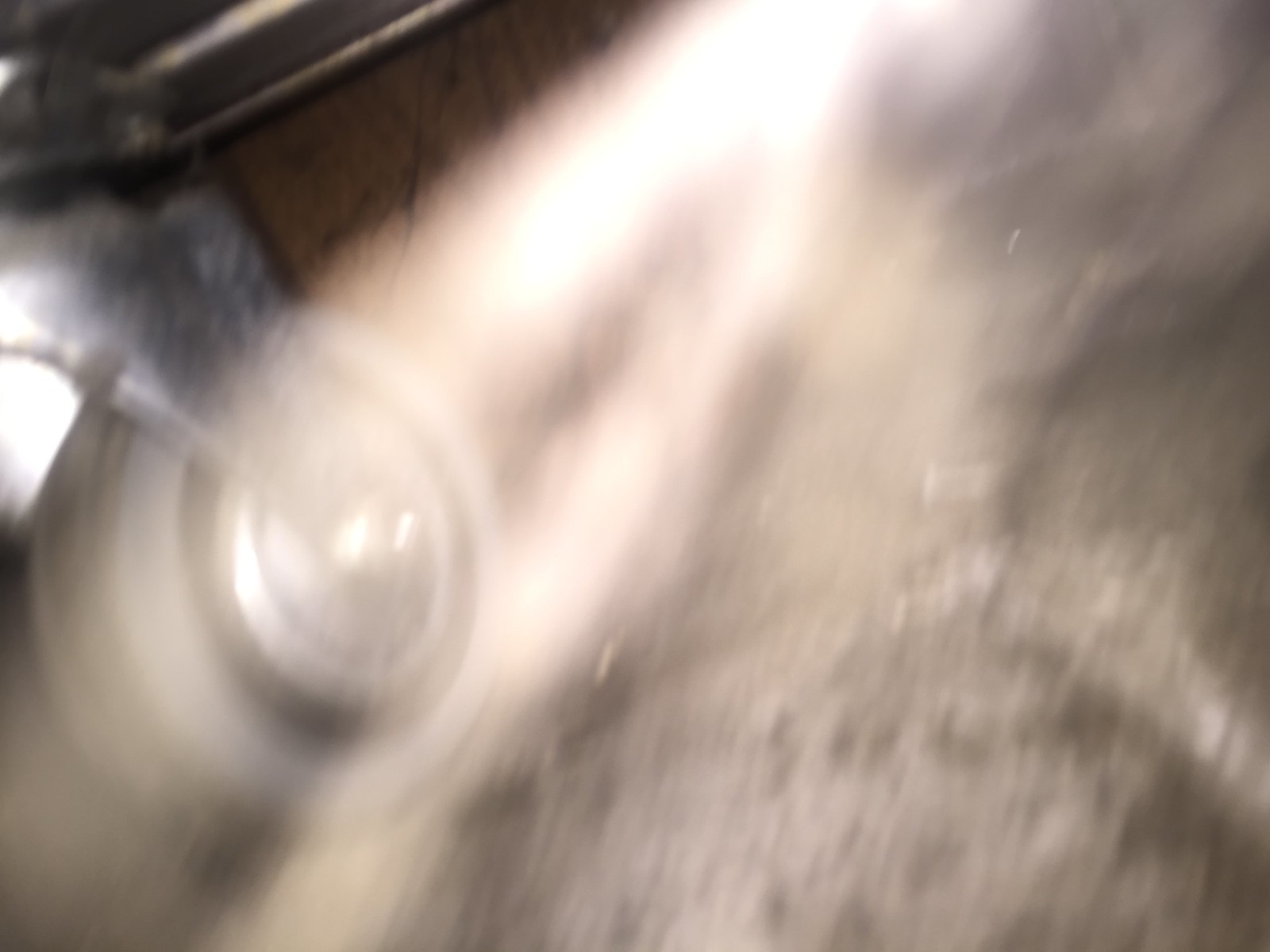The image depicts the interior of a hazy, subterranean bunker. The scene is pervaded by a thick, dusty fog, which diffuses the light shining through from an unknown source, creating an ethereal atmosphere. The floor is made of concrete, contributing to the rugged, utilitarian feel of the space. On the left side of the image, there is a prominent circular object whose details are obscured by the haze. The background is predominantly brown, adding to the murky and aged appearance of the bunker. Overall, the image captures a mysterious, blurry underground setting filled with light and dust.